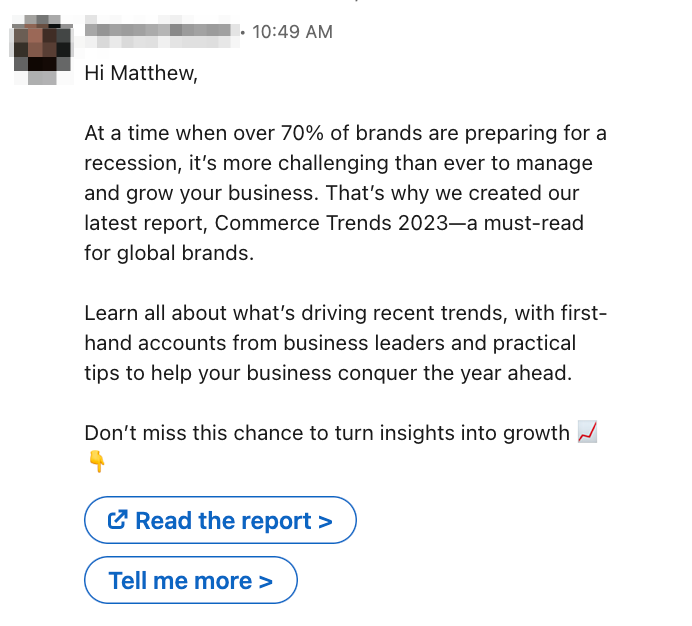The image features a promotional email written at 10:49 AM to a recipient named Matthew, against a white background. The email emphasizes the challenging environment for businesses, citing that over 70% of brands are preparing for a recession. To assist these businesses, the email introduces a detailed report titled "Commerce Trends 2023," which is deemed essential reading for global brands. The report is said to offer insights into current trends, including firsthand accounts from business leaders and practical advice to help businesses grow despite economic challenges.

Prominently displayed in the email are interactive call-to-action elements: 
- A small hand icon with a pointed finger directs attention to a rectangular button outlined in blue that reads "Read the Report." The text is accentuated by arrows, with one box featuring an arrow before the word "Read" and another arrow after "Report."
- Below this, another blue-outlined rectangular button with a right-pointing arrow is labeled "Tell Me More." 

These consistent visual elements encourage the recipient to engage further with the report and related content.